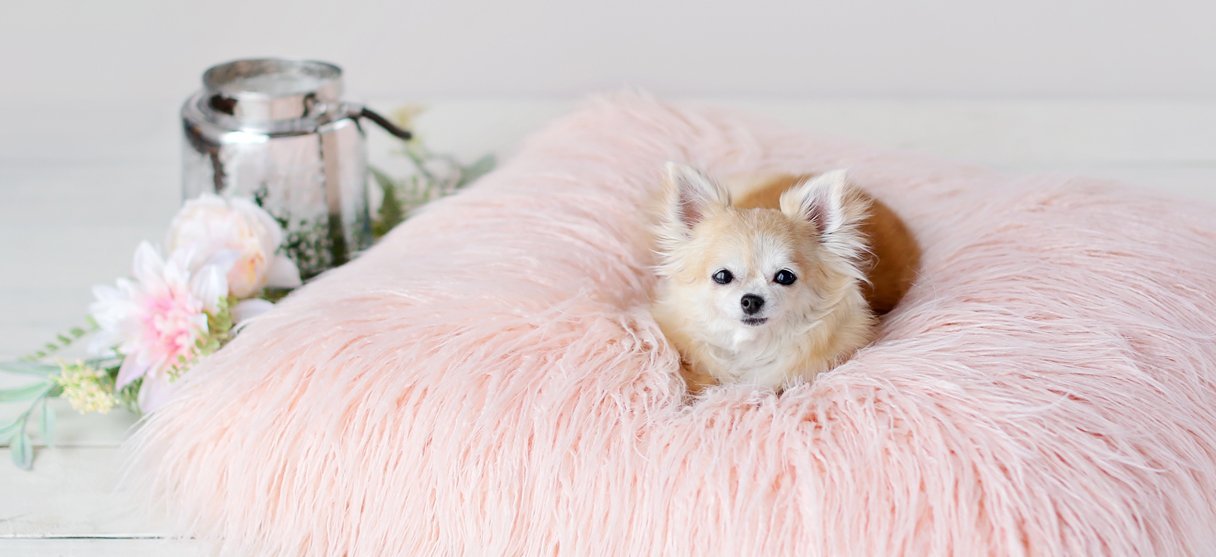This image captures a narrow, horizontal frame of a small dog, likely a Pomeranian or Chihuahua, nestled on a pink, fluffy, feathery-like bed or pillow that occupies much of the lower portion of the photo. The dog sits squarely in the center of this bed, with its tiny legs completely concealed, and gazes directly at the viewer with its beady, black eyes and dark nose. Its fur is a mix of light brown on the face and a richer, darker brown behind, complemented by white eyebrows, beard, and ears. To the left of the bed, there are two flowers positioned in front of a silver metallic cylindrical object. The setting appears to be indoors with a white wall in the background and gray, wood floors beneath the bed, adding a modern touch to the scene.